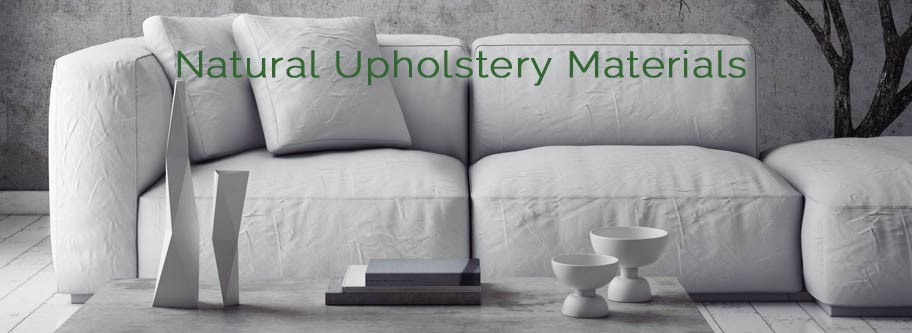The black and white image resembles a furniture catalog and showcases a modern living room with a horizontally cropped, wide composition. Central to the scene is a three-section couch upholstered in light gray material. The couch features two sections with backrests and one with an armrest to the left, while the third section on the right is an ottoman, devoid of backrests, presenting a low, sleek appearance. 

In front of the couch stands a low, white wood coffee table, adorned by two circular bowl sculptures, possibly decorative containers, on the left side. The table also displays a neatly stacked trio of books at its center. To the left of the books, abstract vertical sculptures add a touch of artistic flair to the arrangement.

The backdrop reveals a gray wooden floor and a textured gray wall accented with gray-white trim. A plant with several visible branches occupies the background, its foliage extending beyond the cropped frame, enhancing the natural, indoor setting. The phrase "Natural Upholstery Materials" in green font is prominently displayed at the top center of the image.